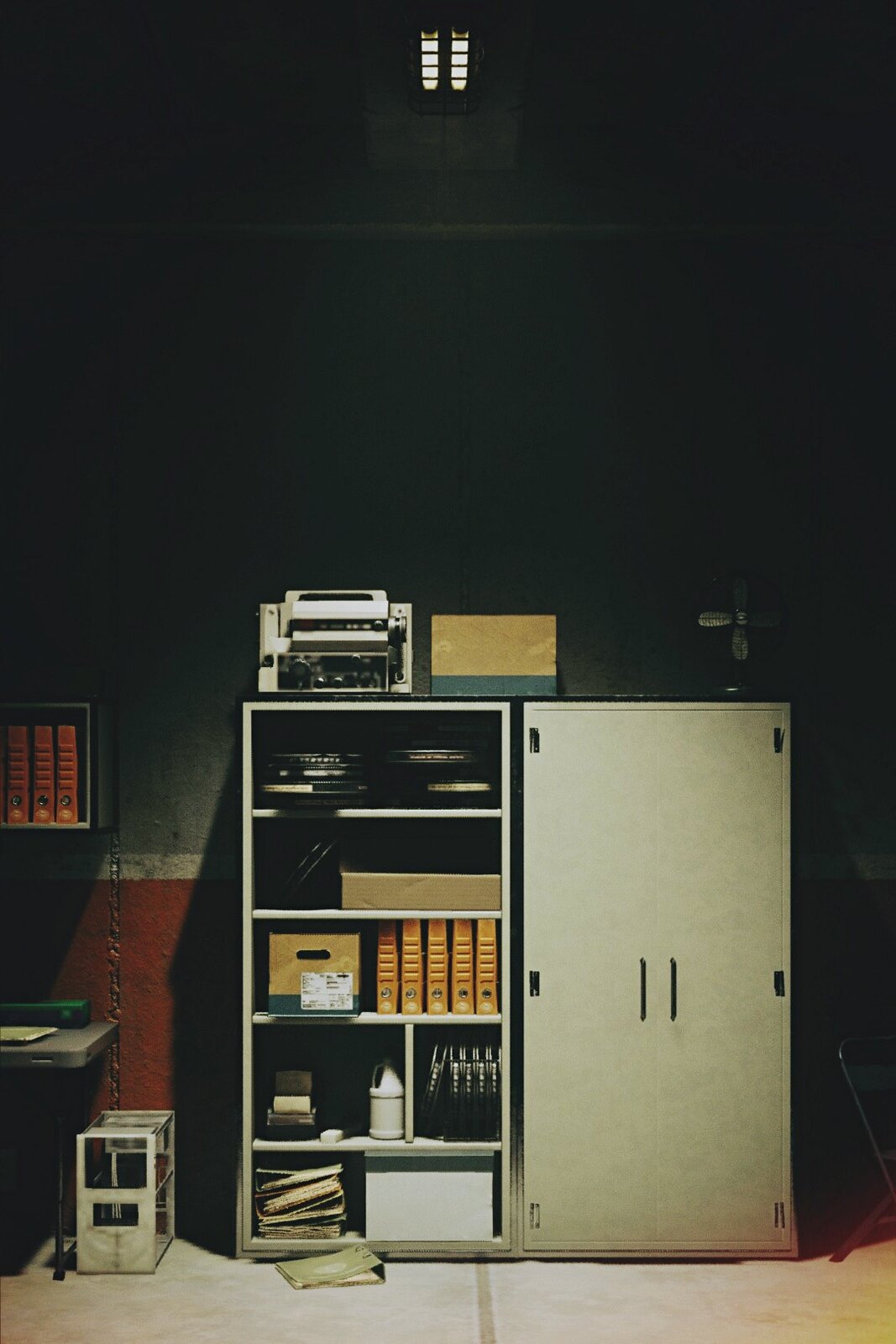The color photograph portrays a dimly lit storage room with several organized shelving units. The gray wall at the back is accented by a horizontal white stripe above a red one, adding a touch of color to the otherwise utilitarian space. 

On the left side of the image stands a bookshelf housing three tall red books with illegible spines. Below it is a gray table with a green item and a white padded envelope placed on top. Adjacent to this table is a small plastic shelving unit.

Dominating the center of the photo is a tall bookshelf with five shelves. The top shelf holds an old printer and a brown cardboard box. The remaining shelves are cluttered with various items, including more red books and several cardboard boxes. There is a white plastic jug and what appears to be an old adding machine among the assortment. A file folder lies on the floor in front of this bookshelf.

On the right side of the image is a tall white storage cabinet. The cabinet's white doors, featuring black handles, are closed, but its top surface is occupied by a black electric fan. This detailed arrangement of objects within the dark room gives an insightful glimpse into a meticulously organized yet densely packed storage area.